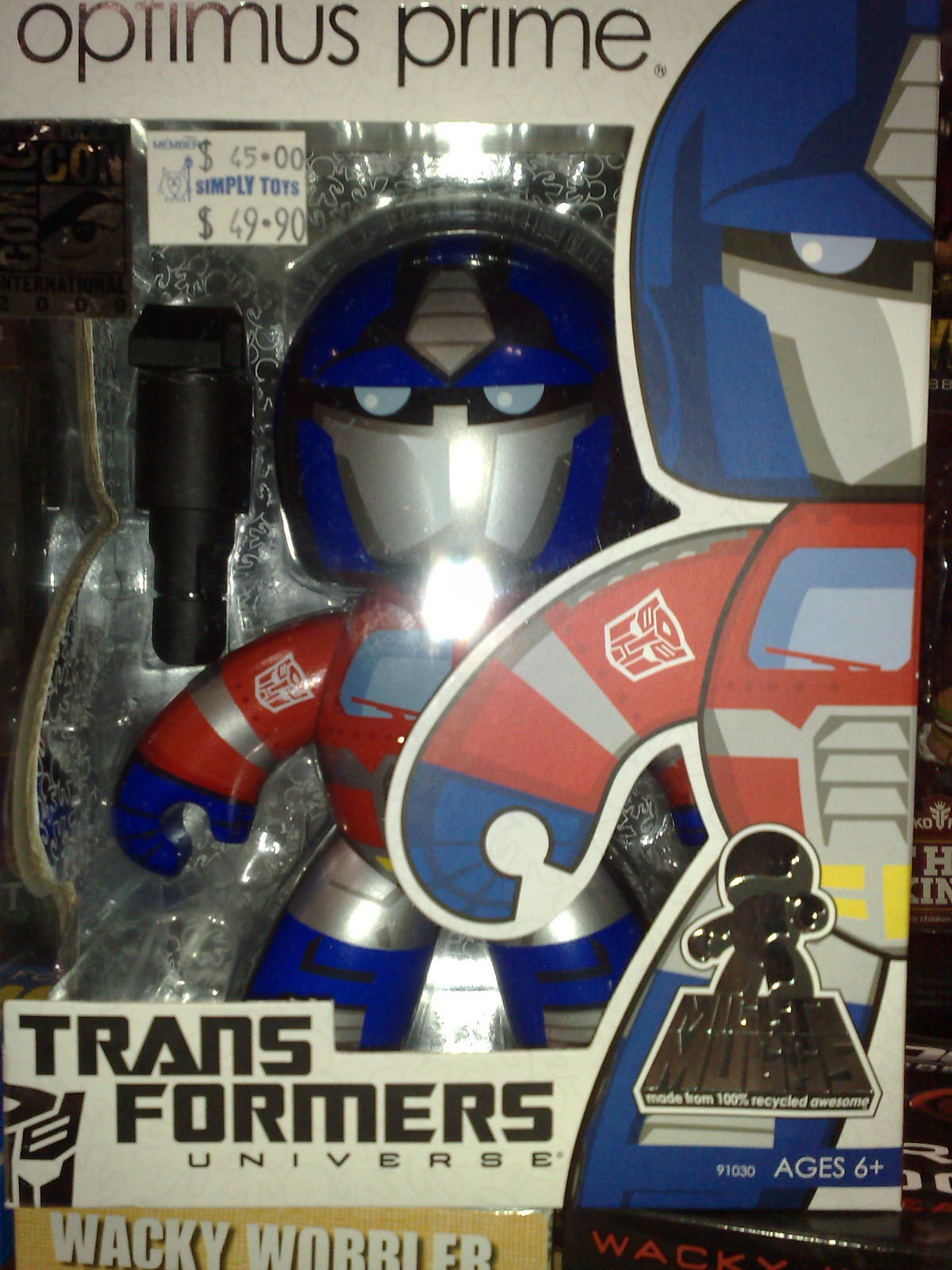This photograph features the front of a toy package for a Transformers figure of Optimus Prime. At the top left corner, a white label bears the name "Optimus Prime" in black font. Just beneath this label is a price tag from Simply Toys, showcasing both a member price of $45 and a general price of $49.90, with a small mascot holding up a light or lantern. The toy, visible through the plastic packaging, displays Optimus Prime with a babyish, rounded design, including a blue helmet, red body, gray torso, and blue hands and feet. Additionally, there's an illustration of Optimus Prime on the right side of the box. At the bottom left corner, the black font reads "Transformers Universe," with "Wacky Wobbler" in white over a yellow bar below it. The recommended age for this toy, indicated at the bottom right, is "ages 6 and up."